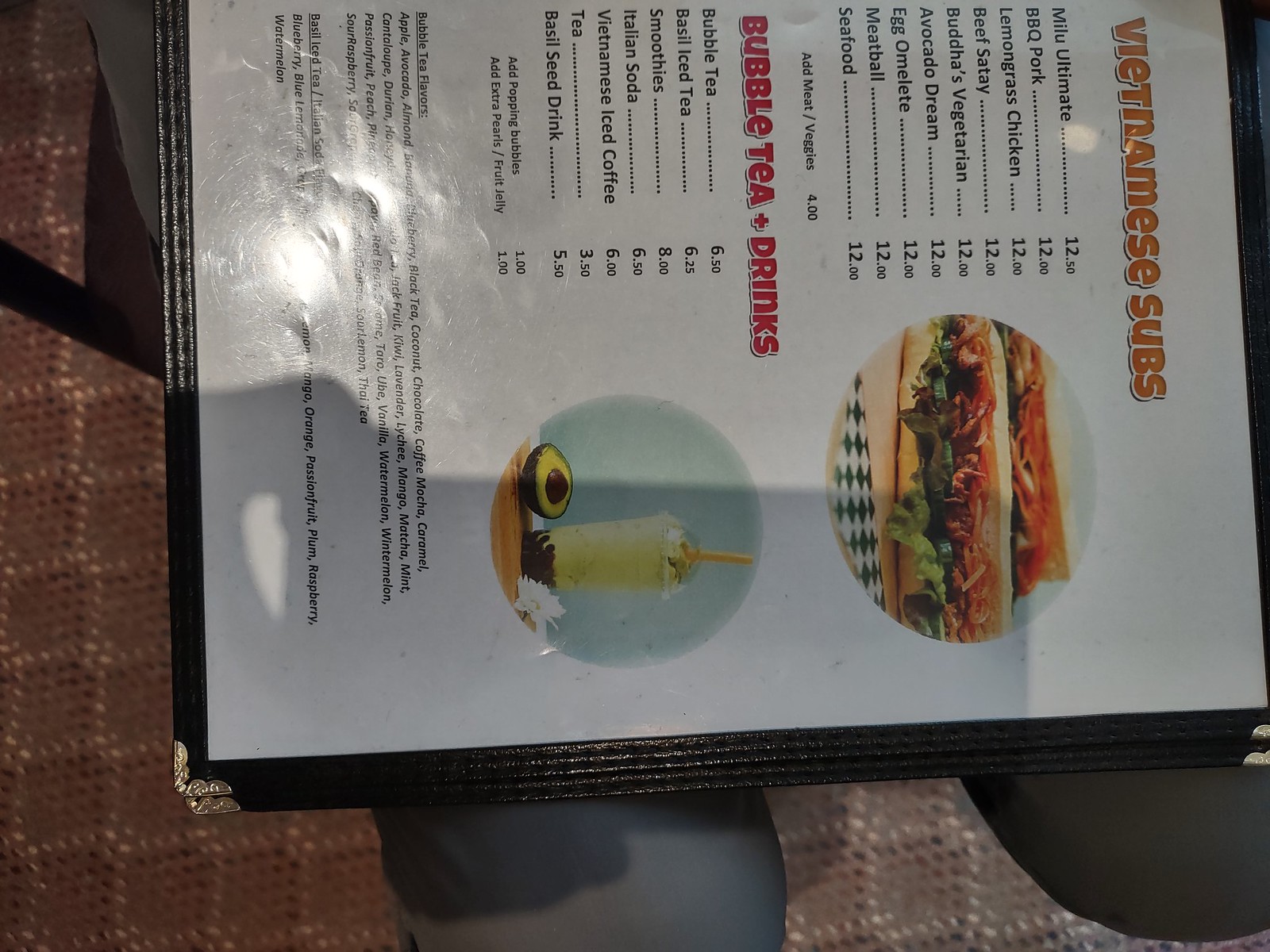The image captures a horizontally rectangular menu page from a Vietnamese restaurant. It is rotated such that the top of the menu is on the right side of the frame and the bottom on the left. The menu is secured inside a menu holder with a black trim and a clear protective cover. 

At the top of the menu, prominently highlighted in orange, the text reads "Vietnamese Subs". Below this title is a list of sandwiches available: 
- Mealoo Ultimate
- BBQ Pork
- Lemongrass Chicken
- Beef Satay
- Buddha's Vegetarian
- Avocado Dream
- Egg Omelette
- Meatball
- Seafood 

Each sandwich on the list has its price indicated to the right. 

Further down (due to the rotation, this appears to the left), there is a circular framed image showing a sandwich filled with various greens. Below the sandwich list, there is a section labeled "Bubble Tea and Drinks", listing various beverages with their corresponding prices. To the right of this drinks list (appearing below due to the rotation), there is another circular framed image of a smoothie in a dome-lidded cup with a straw. Beside the smoothie image, to the left, there is a half of an avocado with its seed facing upwards.